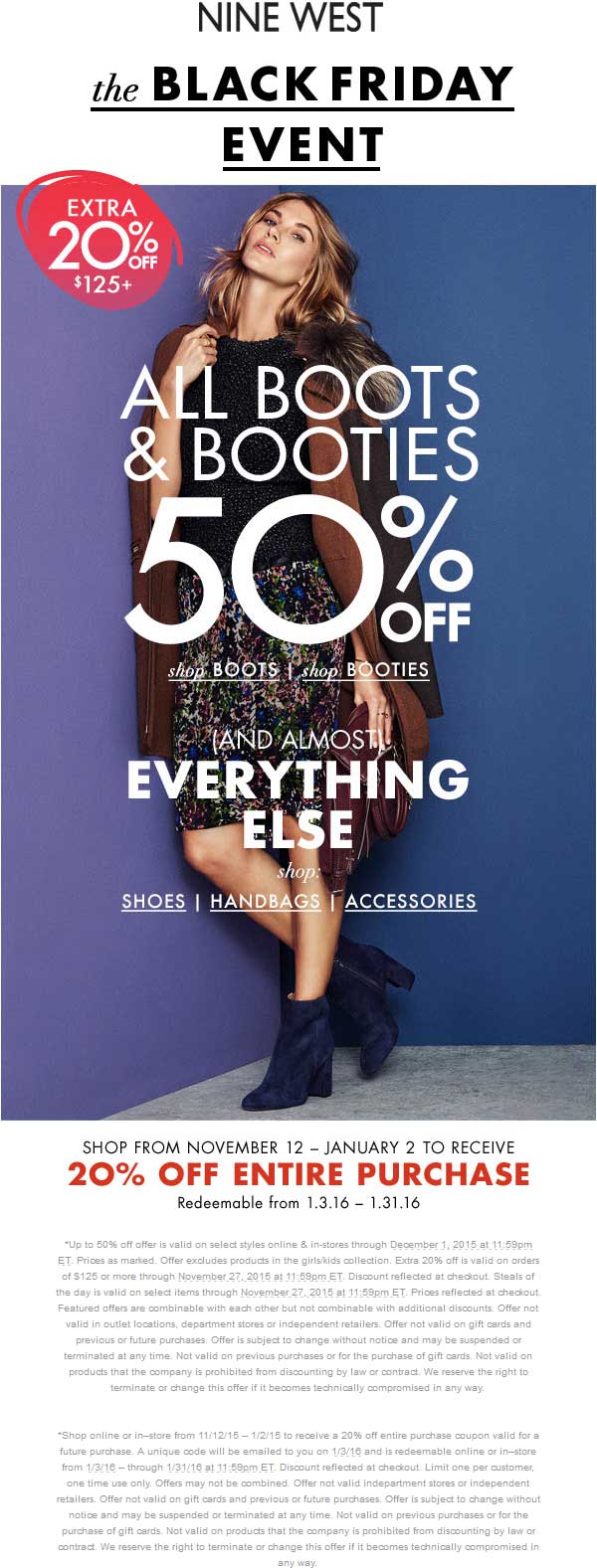In this image, we see a polished advertisement by Nine West. At the top center, the brand's name, "Nine West," is prominently displayed. Directly beneath it, the phrase "The Black Friday Event" is underscored for emphasis. A striking photo of a model dominates the visual, framed by various promotional texts.

In the upper left corner of the picture, a bold red shape catches the eye, adorned with white text proclaiming, "Extra 20% off $125+." Overlaying the image of the model, the main offer is advertised: "All boots and booties 50% off." Additional prompts urge viewers to "Shop boots, shop booties, and almost everything else," followed by an invitation to explore "Shop shoes, handbags, accessories."

Below the model's image is a clean, white background featuring a timeline for the promotion. It reads, "Shop from November 12th to January 2nd to receive," highlighted by "20% off entire purchase" in striking red text. Returning to black font, it clarifies, "Redeemable from 1.3.16 - 1.31.16."

At the bottom, a long list of terms and conditions is meticulously detailed in a smaller, gray-colored font, providing the necessary legal disclaimers and additional information.